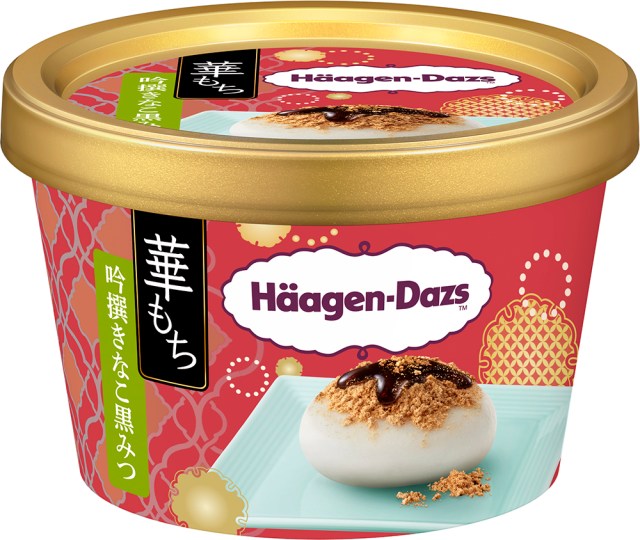The image is a landscape-oriented color photograph featuring a small Häagen-Dazs ice cream container set against a white background. The cylindrical container has a prominent gold-colored band around its lid. The main body of the container is a gradient of light pink and rose colors. The Häagen-Dazs logo is centrally displayed in bold purple letters within a white, oval banner outlined in the same purple shade. Below the logo, there is an image depicting a scoop of ice cream, egg-shaped and resting on a light blue square plate. The ice cream appears to be topped with a crunchy brown topping and drizzled with a brown sauce. To the left of this image, there are two vertical banners containing Asian characters: one black with white text and another green with more white text. The overall design suggests that this is a special edition product likely intended for an Asian market.